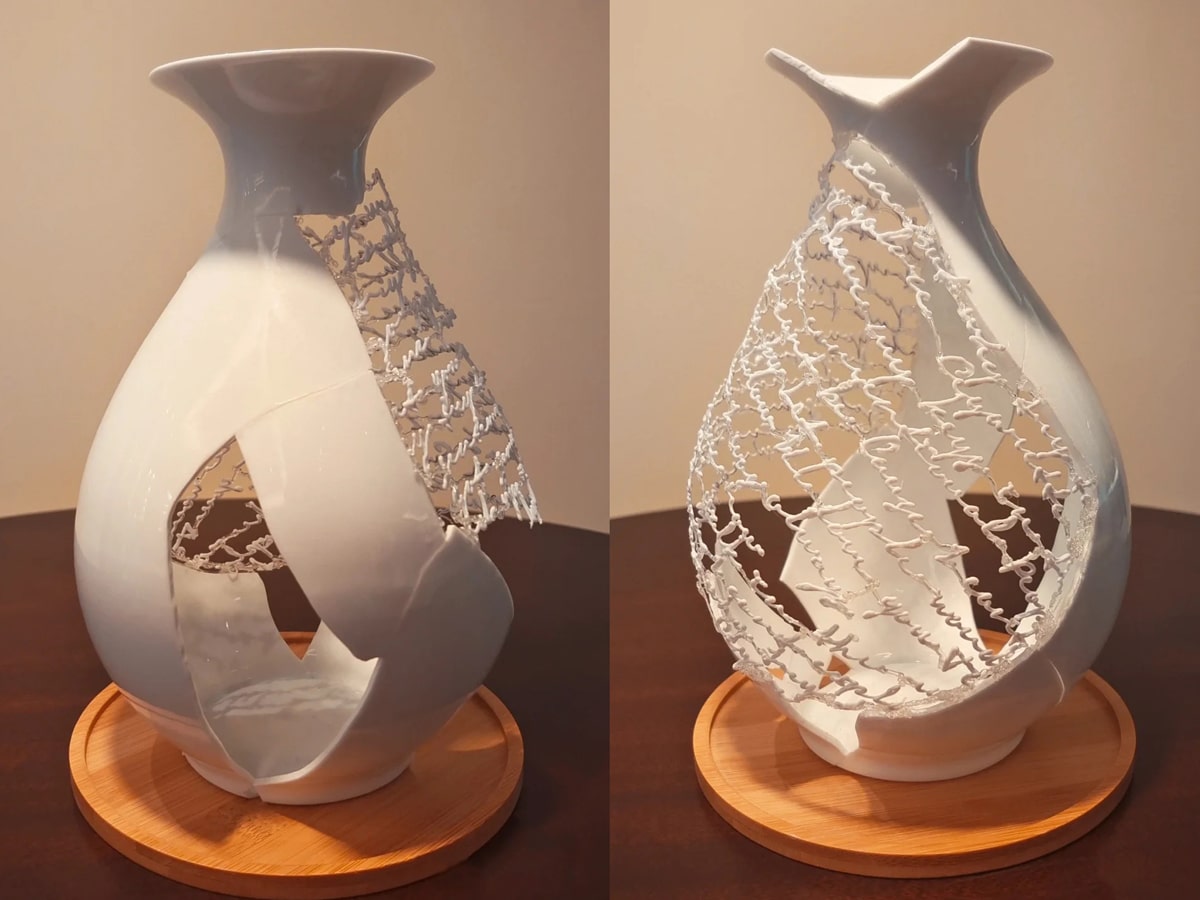The image features a detailed side-by-side view of a highly decorative and intricate white vase, positioned for display indoors. Both images showcase the same vase from different angles, placed on a wooden stand that rests atop a dark brown wooden table. The left image highlights the vase's back, revealing a jagged, cut-open section, which emphasizes its fragile, elegant design. This back portion of the vase consists of delicate ceramic writing, arranged intricately in cursive script. The right image displays the front of the vase, showcasing the continuation of the cascading script that creates gaps throughout its body, allowing a clear view through the vase. The background consists of an off-white or cream-colored wall, enhancing the vase's artistic and abstract appearance. The vase itself has a typical curvy shape, tapering at the bottom and top, but its unique design with text and hollow spaces makes it unsuitable for holding liquid, accentuating its purpose as a piece of art.